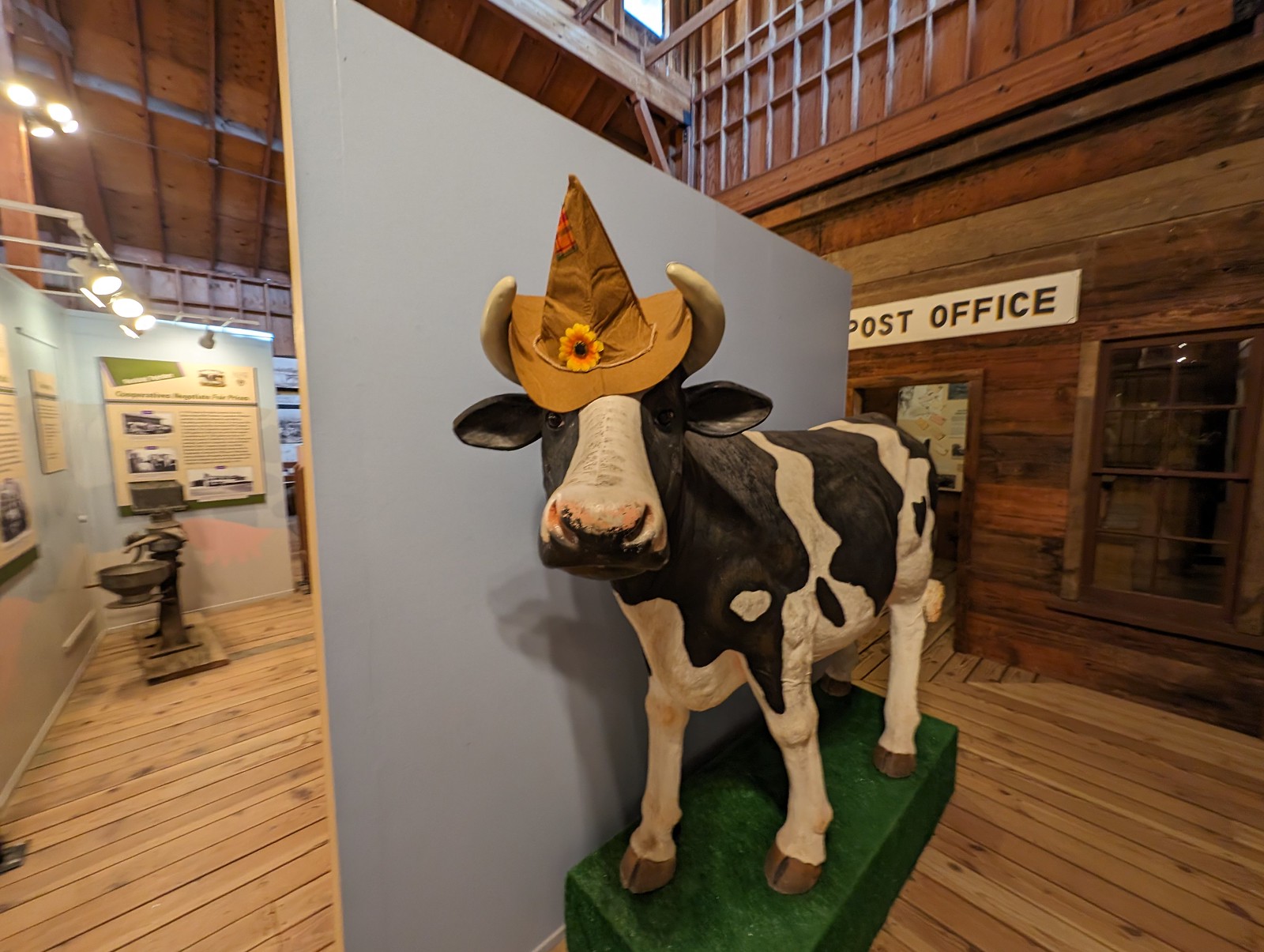This image captures the interior of a museum, specifically a section dedicated to dairy or farm life. Central to the scene is a large black and white cow sculpture, distinguishable by its white face juxtaposed with black patches around its eyes and ears, and small horns. The cow stands on a green platform textured to resemble grass. It is adorned with a yellow pointy hat featuring a decorative white cord, a yellow and orange flower, and an orange patch. The backdrop includes the facade of a wooden post office building, marked by a white sign. The museum's floor, walls, and ceiling are all constructed from light wood, creating a cohesive rustic environment. In the left-hand corner, there is vintage farm equipment accompanied by explanatory posters and spotlights. Additional sections of the museum with informative wall plaques and artifacts can be seen, all illuminated by overhead lighting.